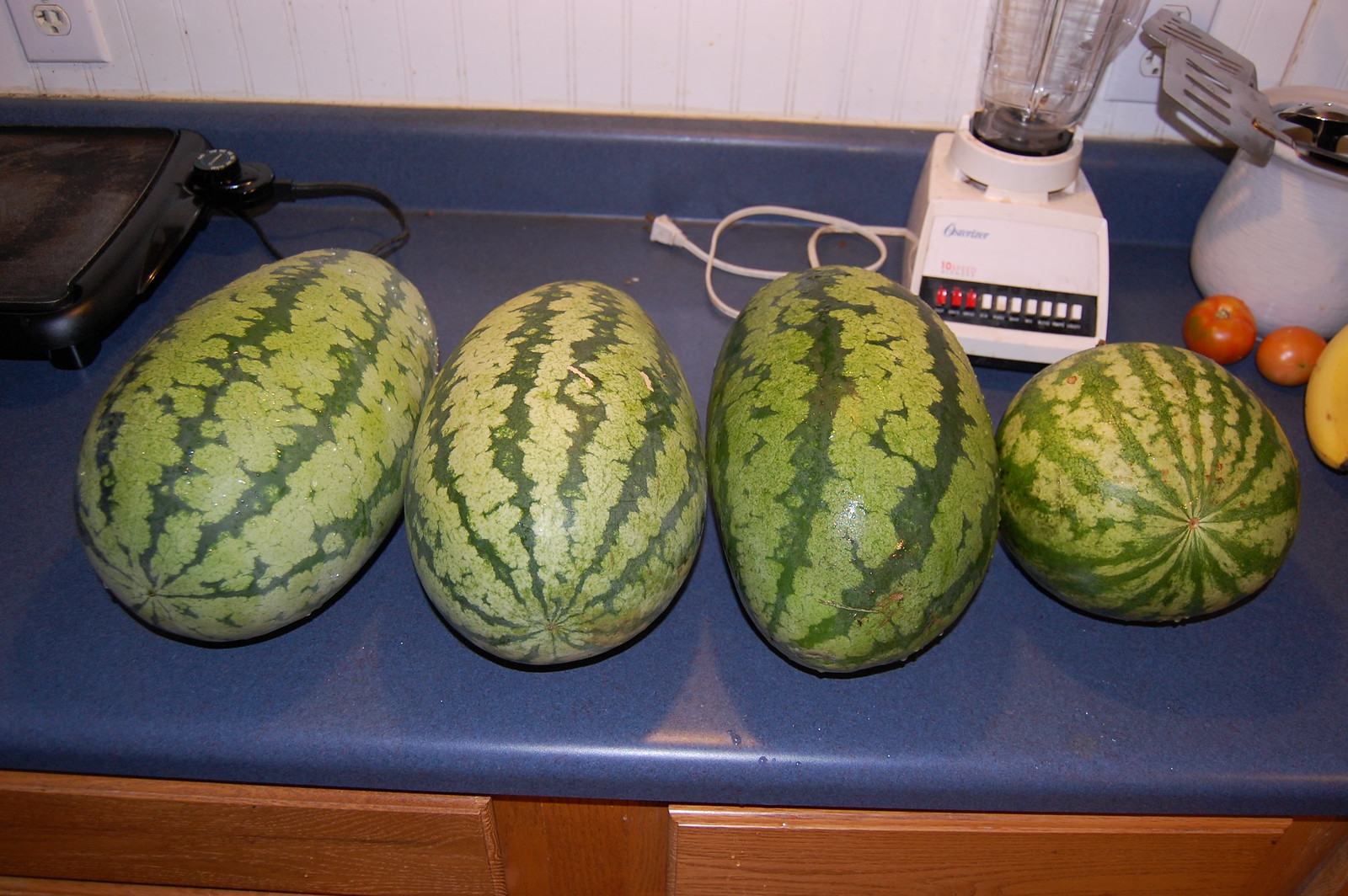The photograph depicts a neatly arranged kitchen countertop with a smooth, dark blue surface and wooden-colored cabinets below. The blue counter is complemented by a blue-black backsplash and a white wall featuring an electrical outlet. On the left side of the counter sits an electric griddle or mini pancake maker, identifiable by its cord trailing down. Prominently displayed in the middle are four watermelons, three of which are oblong, and one is more rounded; all feature dark green and light green striped patterns. Toward the back, an old Oster blender with an array of red and white buttons is positioned just to the right of the watermelons, unplugged, with its cord visible. Adjacent to the blender is a white ceramic utensil holder containing two spatulas and a slotted spoon. Scattered around the counter are two small, red tomatoes and part of a yellow banana, adding a touch of vibrant color to the kitchen scene.